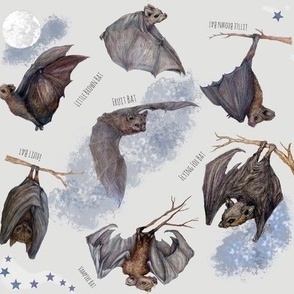This detailed and realistic illustration depicts seven different species of bats, set against a pale grey background. In the top left, there's a depiction of the moon with a blue splotch behind it, emphasizing the nocturnal nature of the scene. Beneath the moon, a bat with its wings stretched upward is in mid-flight. Slightly to the right and up, another bat in flight has its wings stretched downward, its grey form contrasting against the background. Further right, a branch extends from the edge of the frame with a bat hanging upside down, its wings wrapped around its body, and accompanied by some indecipherable text and an angled blue star above the branch.

At the center of the illustration, a labeled "Fruit Bat" spreads its wings wide like a plane, with another blue splotch behind it, making it the focal point. Below it to the left, another branch extends with a bat hanging down, its body cocooned within its wings; stars forming the Big Dipper constellation are depicted beneath this bat. In the bottom center, several branches appear to hang in mid-air with yet another bat hanging upside down, its grey wings partially folded and accompanied by more indecipherable text nearby. Finally, in the bottom right, a bat hangs from yet another branch, its wings held halfway out as it peers up towards the observer, framed by a blue blotch and additional hard-to-read text to the left.

The image is speckled with stars and color blobs to symbolize the night sky and is likely intended as an educational piece, despite some of the text being difficult to read. The bats are illustrated in lifelike detail, with some in flight and others hanging from branches, providing a comprehensive overview of their various poses and appearances.